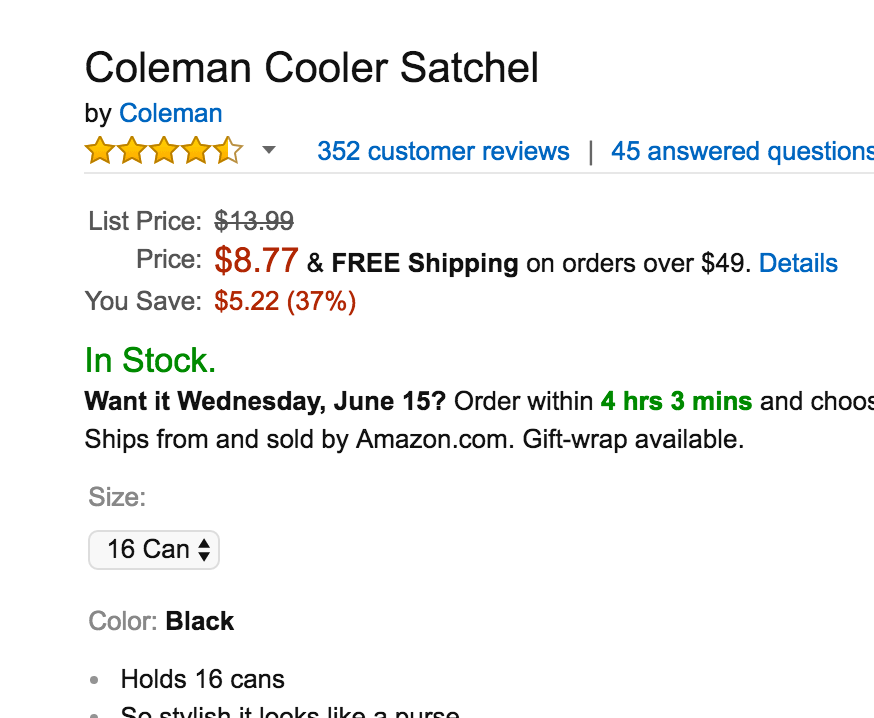The product image depicts a Coleman Cooler Satchel available for purchase on a website resembling the layout of Amazon. 

In the upper left corner, the item is labeled "Coleman Cooler Satchel" in bold, black text. Below, it reads "Buy Coleman," with "Coleman" presented as a clickable blue link.

The product boasts a rating of 4.5 stars from 352 customer reviews and has 45 answered questions. The list price of $13.99 is shown, but it is crossed out to highlight the current sale price of $8.77. The offer includes free shipping on orders over $49, with detailed information available through a link. Purchasing at the sale price saves the buyer $5.22, which is a 37% discount.

The item is in stock and can be delivered by Wednesday, June 15, if ordered within four hours and three minutes. It is shipped from and sold by Amazon.com, and gift wrapping is an available option. 

The cooler is sized to hold 16 cans and comes in a stylish black color. Its design is sleek and fashionable, resembling a purse.